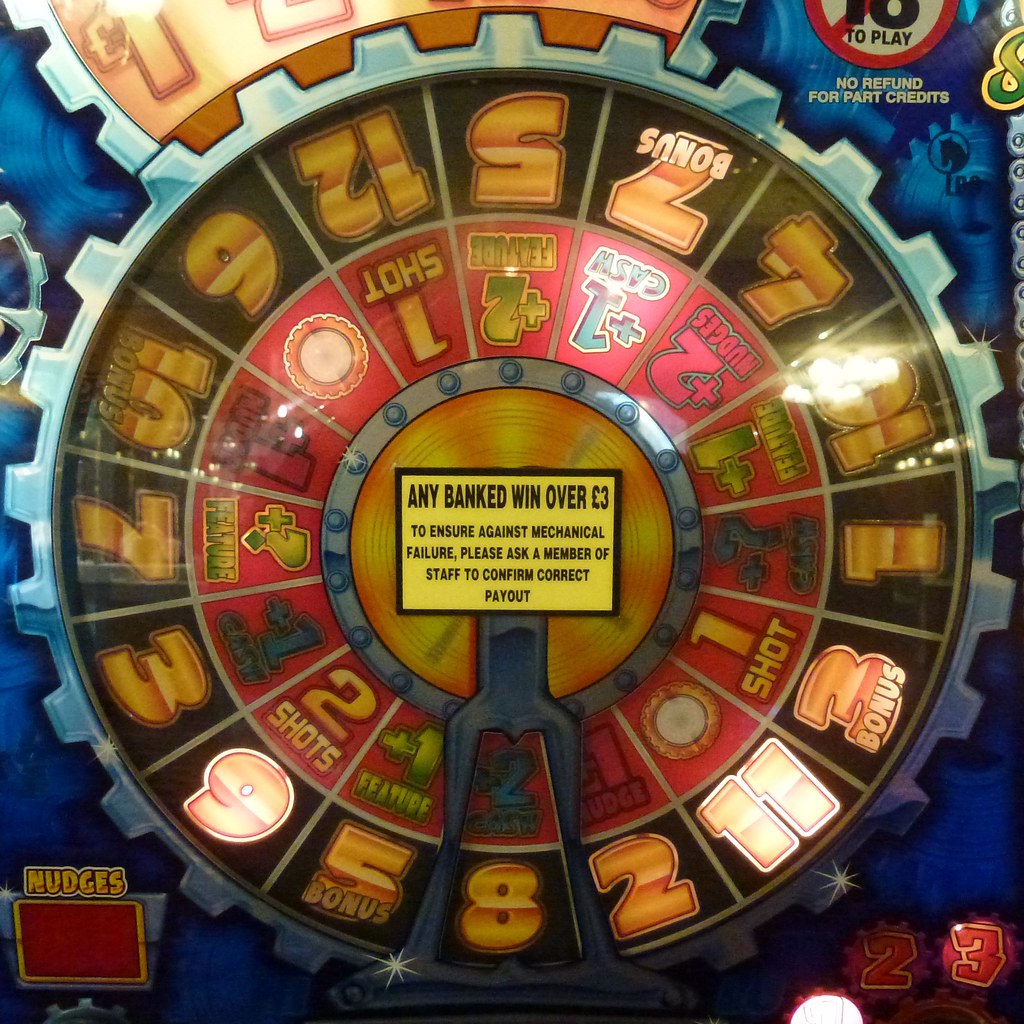The photograph depicts an intricately designed casino game featuring a multi-tiered wheel with illuminated sections. The outer edge of the wheel is designed to resemble mechanical gears and displays gold-colored numbers, some of which—such as 7, 11, 3, and 6—are currently lit. Inside this gear-like rim, a red wheel contains sections labeled with commands like "one shot," "two shots," and "plus two shots," as well as bonuses. The inner part of the wheel includes more colorful sections and commands like "plus 2 nudge," "plus 1 cash," "7 bonus," "5," "12," and "6." A noticeable element in the center of the wheel is a yellow sign with black text stating: "Any banked win over three British pounds to ensure against mechanical failure, please ask a member of the staff to confirm correct payout." The overall appearance is that of an engaging casino or arcade game with vivid lights and various gambling incentives.